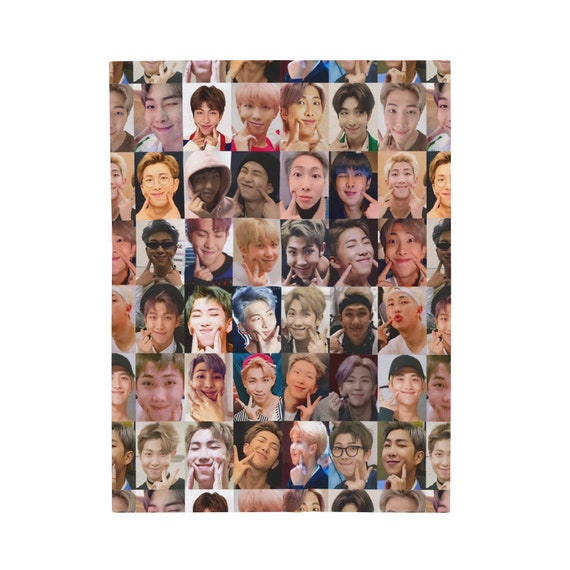This image is a meticulously arranged rectangular collage featuring numerous faces of likely the same individual of Asian ethnicity, possibly Japanese, given their varied hairstyles and appearance. The collage, which spans about eight rows (with parts cut off at the top, bottom, and sides), portrays the person in different hairstyles—ranging from multicolored locks like pinks and browns to a few shots with blonde hair. In each photo, the individual is smiling and making peace signs or touching their cheeks with their fingers in various poses, resembling a dynamic array of yearbook photos. The variations in hair color, poses, and expressions make each image distinct while retaining a cohesive theme through the repetitive portrayal of the same individual.